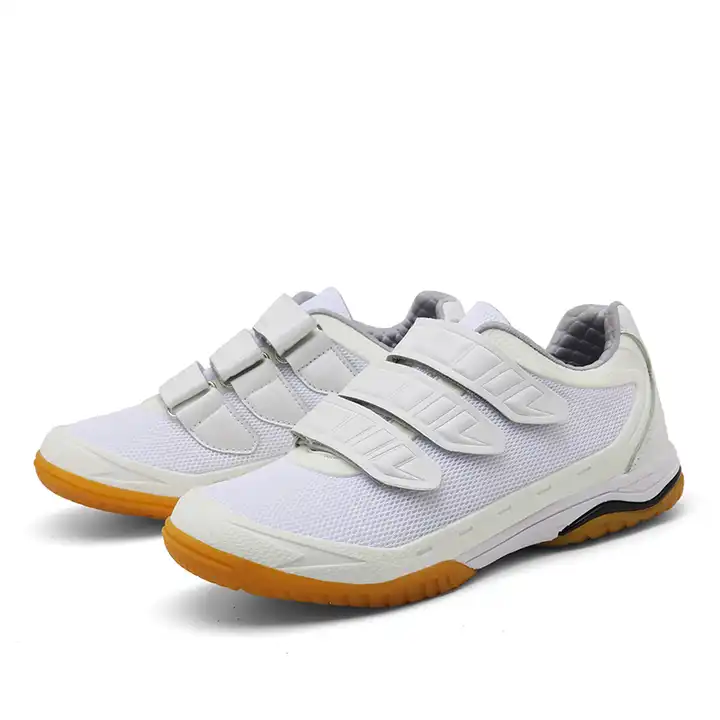This photo showcases a pristine pair of white tennis shoes, commonly known as sneakers or gym shoes, staged on a white surface with a matching white background. These new, immaculately clean shoes feature three Velcro straps for convenient fastening, making them suitable for individuals who may struggle with traditional laces, such as older adults with arthritis. 

Each shoe is detailed with yellow and black soles made of brown rubber, providing a sturdy foundation. The interior of the shoes around the heel is lined in gray, and a gray line runs from the back of the heel towards the start of the Velcro straps. Additionally, a white band wraps from the toe along the side to the back of the shoes. The breathable material on the shoe's upper and the rubber material surrounding the toe area highlight a thoughtful design for both comfort and durability. The shoes are positioned side by side, with the left shoe slightly in front and closer, allowing a detailed view of the left side and front of the right shoe, perfect for an advertisement showcasing their features.